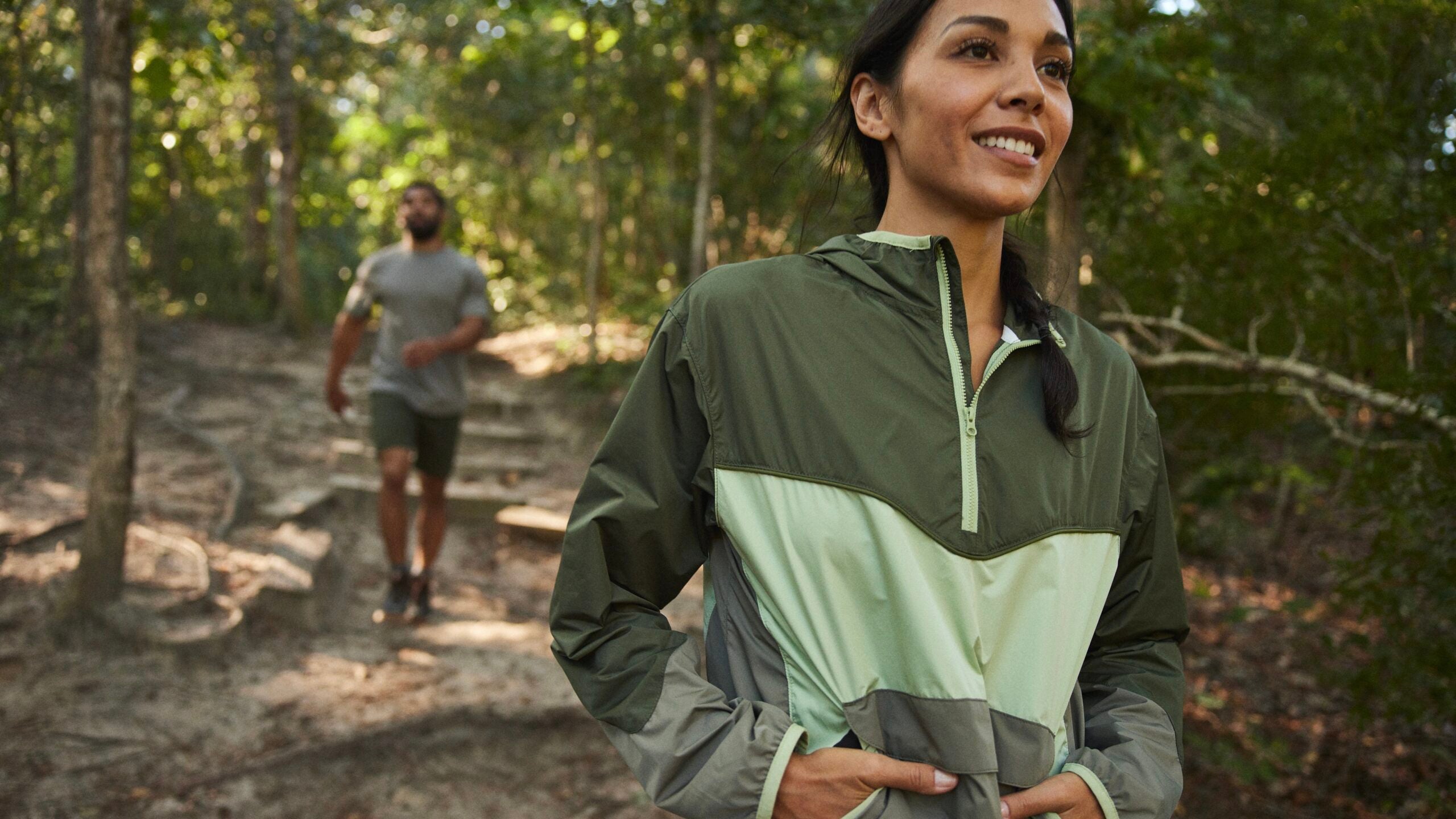A full-color, horizontally rectangular photograph captures an outdoor scene on a sunny day, suggesting professional quality with no border. Set in a wooded area with thick green vegetation, a dirt trail with square log steps extends through the center of the image. Sunlight filters through the tree canopy, casting dappled light and shade across the path and through the leaves, revealing a glimpse of blue sky.

In the foreground stands a young woman with dark, shoulder-length hair and dark brown eyes. She smiles brightly, her hands mostly in the pockets of a quarter-zip windbreaker that features stripes of dark gray, beige, and lighter gray. The sage and mint green hues of her jacket blend subtly with the natural surroundings. Her thumbs are visible outside her pockets as she looks toward the right of the image.

In the background, a man in olive shorts and a gray t-shirt descends the steps, though he appears blurred, making it difficult to discern specific details about him. The overall composition emphasizes the serene forest setting, punctuated by the natural sunlight and the joyful presence of the woman in the foreground.